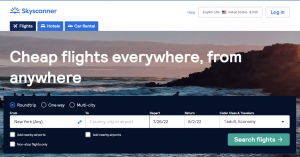This is a detailed and descriptive caption for the image:

The screenshot captures a webpage from a flight booking website, Skyscanner. The layout includes a blurred yet identifiable blue header spanning the top. Below the header is the Skyscanner logo, accompanied by a small symbol, and to the right, the partially legible word "Help." Adjacent to this is a search bar featuring an American flag and some indistinct text. 

Below the search bar, a white button marked "Log In" in blue text is visible. The page offers three interactive options: "Flights," "Hotels," and "Car Rental." The "Flights" option is highlighted in a darker blue, indicating it is currently selected, while the other two options are in a lighter blue.

Dominating the main section of the image is a scenic photograph showing water, sky, and rocks. Superimposed on the photo is the text "Cheap flights everywhere, from anywhere" in white typography. Below this tagline is a prominent white rectangular input box designed for entering flight details, though its text and numbers are too blurred to decipher.

At the bottom right corner of the image, a green rectangular button with the inscription "Search Flights" in white, accompanied by a white arrow, is positioned, inviting users to proceed with their flight search.